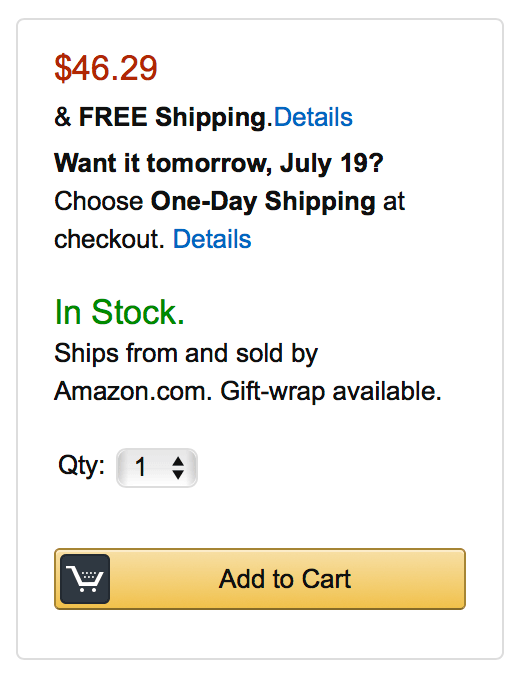This image showcases a segment of a website, specifically a product listing page. Dominating the page are the large numbers "4629," indicative of a price or an important numerical feature. Directly beneath these numbers, the phrase "Free Shipping" appears in black text, accompanied by "Details" in blue, suggesting a hyperlink for additional information.

A section asks, "Want it tomorrow, July 19th?" followed by a prompt to "Choose One-Day Shipping at checkout," with "Details" again highlighted in blue, providing a consistent user experience.

The stock status is prominently displayed in large green letters stating "In Stock." Below this, the text "Ships from and sold by Amazon.com" clarifies the product's origin and seller, reassuring potential buyers. A note also mentions that "Gift-wrap available."

Under the quantity section, the default selection is "1." At the bottom of the page, a distinct orange bar features the "Add to Cart" button, a fundamental e-commerce call to action. To the left of this button, a black square icon with a graphic of a white cart speckled with dots hints at shopping cart functionality.

The overall webpage layout is minimalist, with a white background framed by a thin gray border, keeping the focus on product details. Despite the absence of explicit Amazon branding, the narrative and color scheme – specifically the use of orange, gold, and black – unmistakably align with Amazon's familiar design elements.